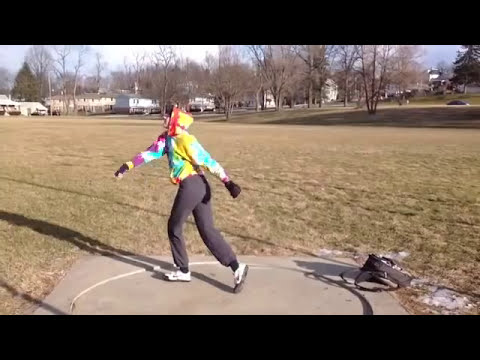The image depicts a person, likely a white male, practicing a throw—possibly shot put or hammer throw—within a small, square cement area that has a circular section etched into it. The individual is outfitted for cold weather in a tie-dye hoodie with shades of white, yellow, and red, paired with gray sweatpants, white sneakers, and black gloves. Positioned facing left with outstretched arms and legs apart, as if captured immediately after executing a throw, the figure is surrounded by a park setting. A black backpack lies on the ground in the bottom right corner of the image. In the background, an expansive field with short, greenish-brown grass stretches out, bordered by a row of trees devoid of leaves, suggestive of winter. Distant residential houses can be seen along the top left, set against a partly cloudy sky with hues of blue and white.